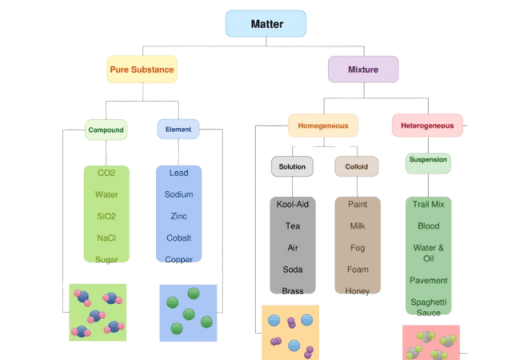The image depicts a detailed and colorful diagram classifying matter into several categories. At the top, matter is divided into pure substances and mixtures. Pure substances are further categorized into elements and compounds, with examples of compounds including CO2, water, SeO2, NaCl, and sugar, and examples of elements including lead, sodium, zinc, cobalt, and copper. Mixtures are divided into homogeneous and heterogeneous types. Homogeneous mixtures are further subdivided into solutions and colloids, with solutions including examples such as Kool-Aid, tea, air, soda, and brass, and colloids including paint, milk, mist, foam, and honey. Heterogeneous mixtures include suspensions, with examples such as trail mix, blood, water and oil, and spaghetti sauce. The background of the diagram is a plain white, making the colorful categories stand out clearly.